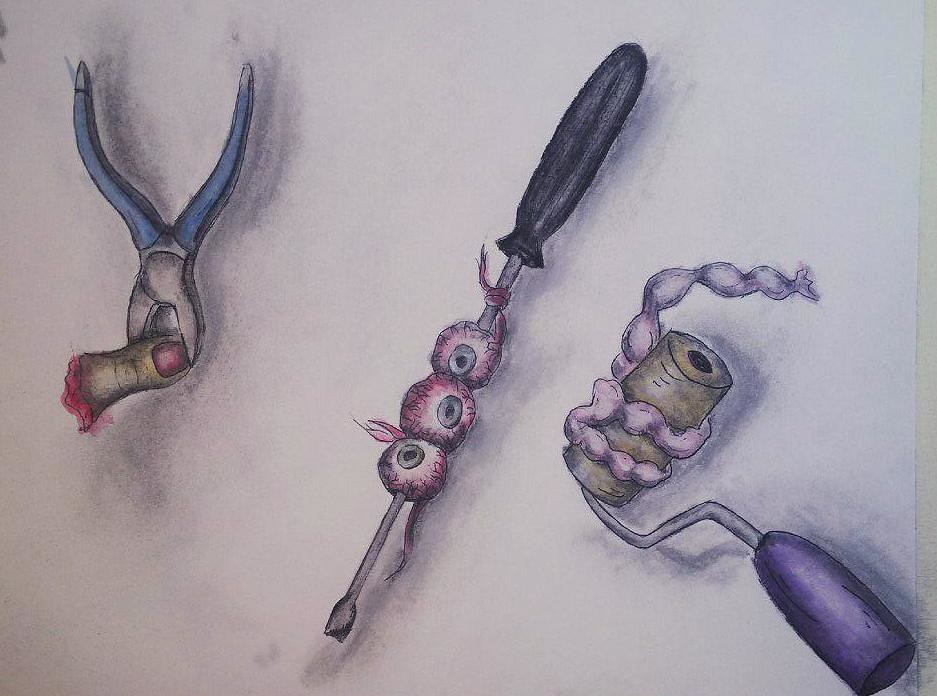The artwork portrays a stark, grisly scene set against a gray background, focusing on a collection of vividly illustrated tools. Dominating the upper left quadrant, a pair of pliers with blue handles grips a severed finger, the working area of the pliers rendered in metallic gray. The finger itself boasts a red-painted nail, with a grotesque, bloodied stump just below the first knuckle, exposing visceral details of the injury.

Centered in the composition, a menacing screwdriver stands erect. It features a black handle and an extended gray shaft. Intertwined along the shaft are three disembodied eyeballs, each eerily lifelike with gray irises, black pupils, and a mix of red and white sclera. The top eyeball is secured with a red string, adding an unsettling touch.

In the lower right corner, a paint roller completes the macabre display. It sports a black handle extending into a gray rod leading up to the roller itself, which is unnervingly wrapped in what appears to be human intestines, emphasizing a theme of human craftsmanship intertwined with horror.